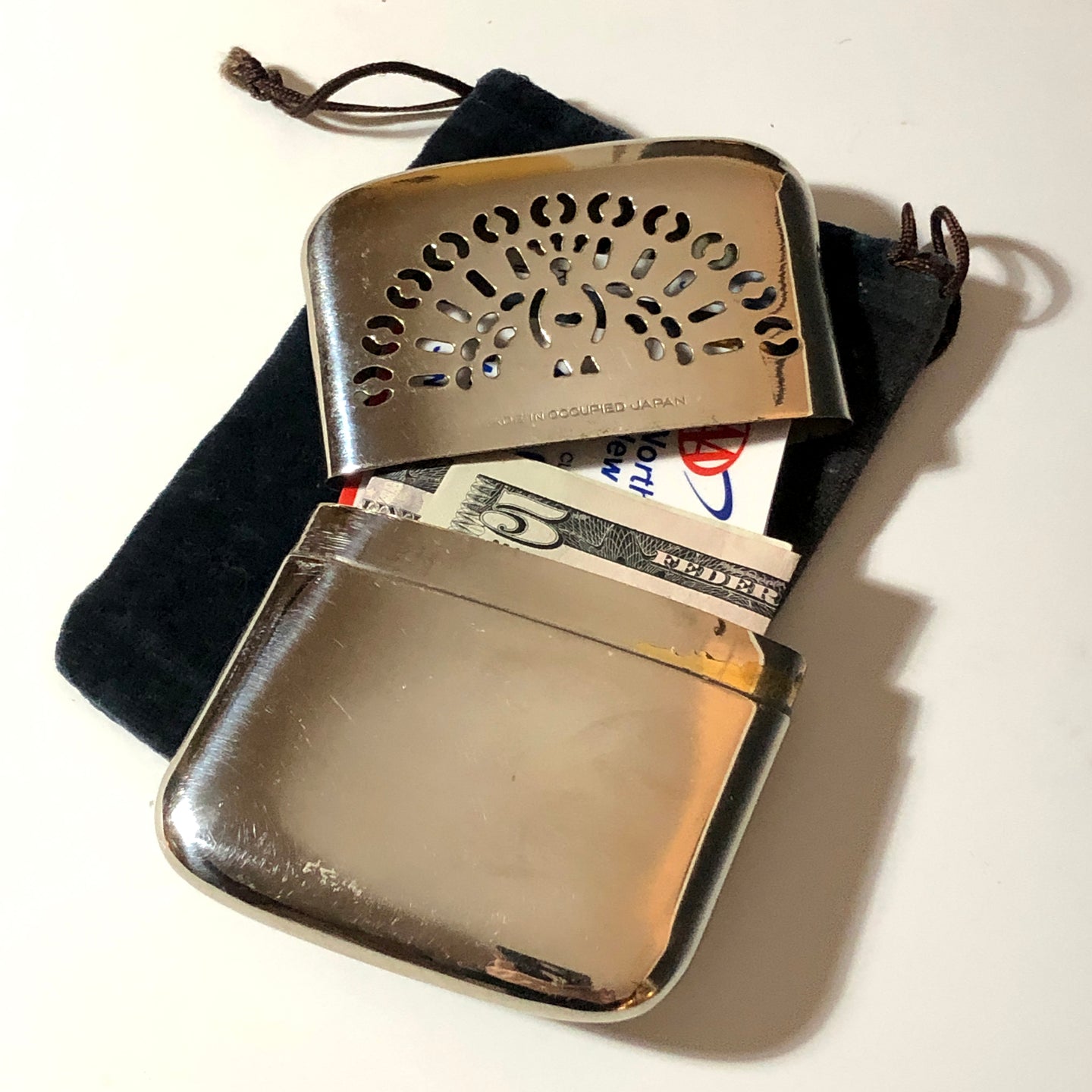This is a detailed indoor photograph showcasing a unique metal pocket holder, often mistaken for a cigarette lighter due to its appearance. The item is crafted from tinplate, bearing decorative curved perforations on its top lid, mimicking ventilation holes typically found in lighters. Engraved on this lid are the words "Made in Occupied Japan." The lower compartment of the holder is solid silver with no perforations, seamlessly sliding over the contents inside.

Within the pocket holder, there's a visibly folded five-dollar bill labeled with "five" and "federal," along with a AAA card, displaying the letters "A," "A," "O," "R," "T," and "W." The compact metal wallet sits atop a black velvet pouch with a drawstring, casting a distinct shadow against a cream-colored background. The light source is positioned to the left of the frame, further enhancing the shadow's dark gray hue and the intricate details of the metallic holder.